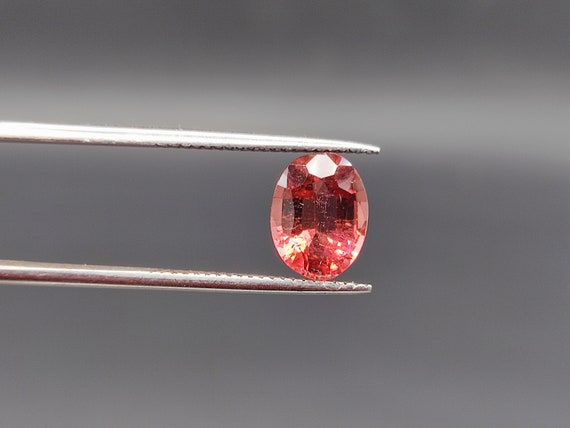In this highly detailed close-up image, a pair of precision needle-nose tweezers with finely pointed tips grasps a vibrant red gemstone. The tweezers emerge from the left center of the frame, their metallic surface gleaming subtly under soft lighting. The background features a dark gray tone, contrasted by a faint white horizontal line running through the upper portion, adding depth to the composition. The focus is tightly held on the gemstone, obscuring the full length of the tweezers and highlighting the meticulous grip on the jewel.